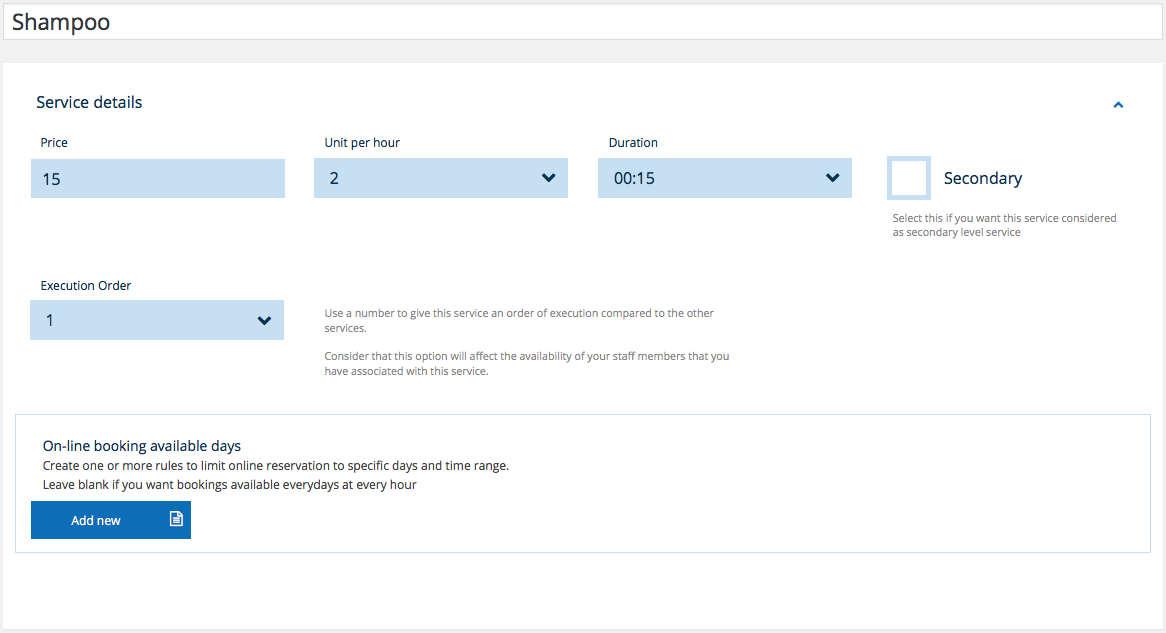**Detailed Caption:**

The image displays a web page or application screen dedicated to configuring a service labeled "Shampoo." The service details are broken down as follows: 

- **Price:** $15
- **Units per Hour:** 2
- **Duration:** 00:15 (which could be interpreted as either 15 seconds or 15 minutes, although 15 minutes is more likely)
- **Execution Order:** 1 (A note next to this field explains that you should use a number to indicate the order of execution for this service in relation to others. It also cautions that this setting will affect the availability of staff members associated with this service.)

Further down, there’s a section for "Online Booking Available Days" where the user can create rules to limit online reservations to specific days and time frames. If left blank, bookings are available every day at all hours.

At the bottom of the page, there is a blue button with a white paper icon labeled “Add New,” presumably for adding a new service or rule.

This interface is designed to help users manage the scheduling and execution of services efficiently, ensuring clarity and precision in staff availability and customer bookings.